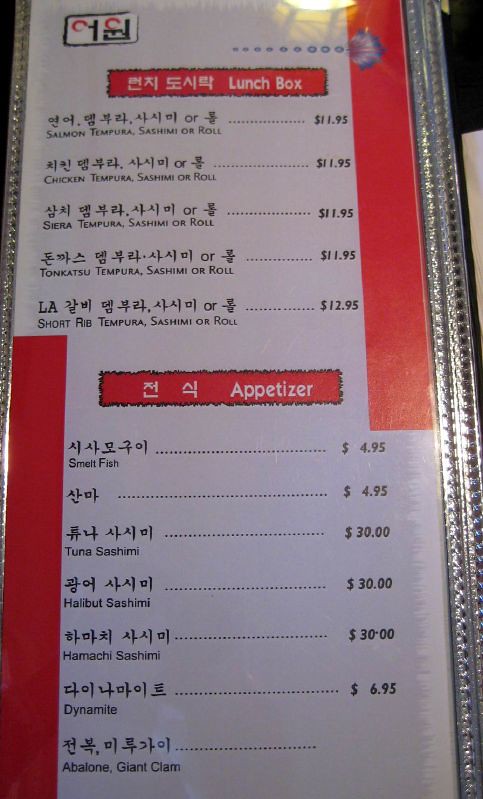This image showcases a Chinese menu with a distinct and clean design. The menu's background is predominantly white, accented with a striking red trim. Section headings stand out with their red background, black borders, and white text, creating an organized and visually appealing layout. 

The first section at the top is labeled "Lunch Box." Each item in this category is presented in Chinese, followed by its English translation. The menu items include a variety of tempura options such as salmon, chicken, tonkatsu, and short rib.

Directly beneath the Lunch Box section, the Appetizer menu is displayed. This section lists items such as small fish, tuna sashimi, halibut sashimi, hamachi sashimi, dynamite, abalone, and giant clam. The names of the dishes are aligned on the left side of this section, while the prices are clearly indicated on the right. Each dish name is followed by its English translation below the Japanese script, ensuring clarity for all customers.

Overall, the menu is well-organized with a neat, clear structure that makes it easy for diners to navigate and choose their desired dishes.